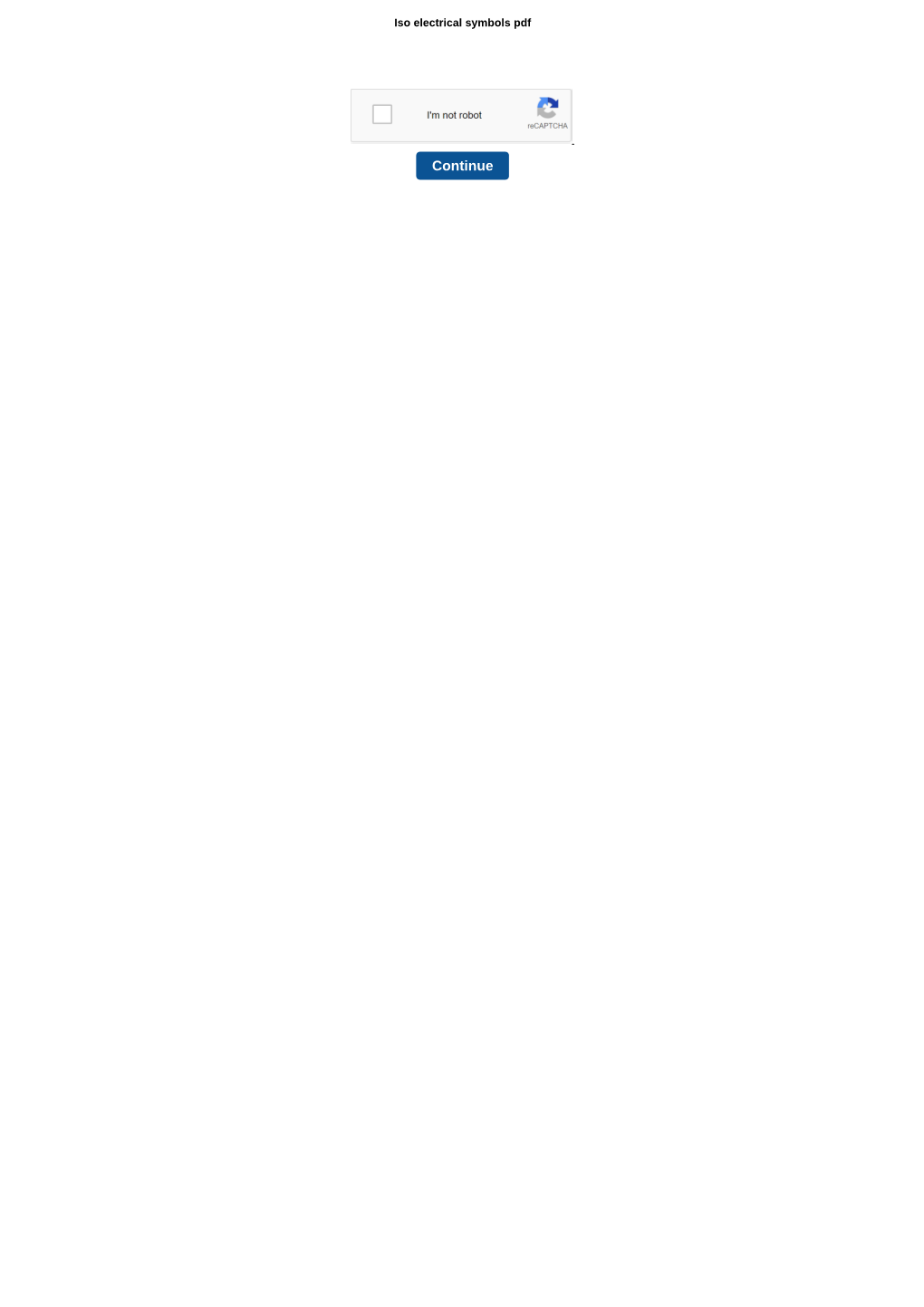The image features a document with a white background, seemingly titled "Electrical Symbols PDF," though the text is somewhat small and difficult to read. Dominating the lower portion of the image is a gray rectangle containing a checkbox labeled "I'm not a robot." Adjacent to this checkbox is a circular arrangement of three arrows in varying shades: gray, light blue, and dark blue, identified as the reCAPTCHA logo. Below this, a prominent blue rectangle appears with the word "Continue" written in white capital letters, prompting further interaction. The overall design elements suggest a user verification process, likely as part of an online form or download action.